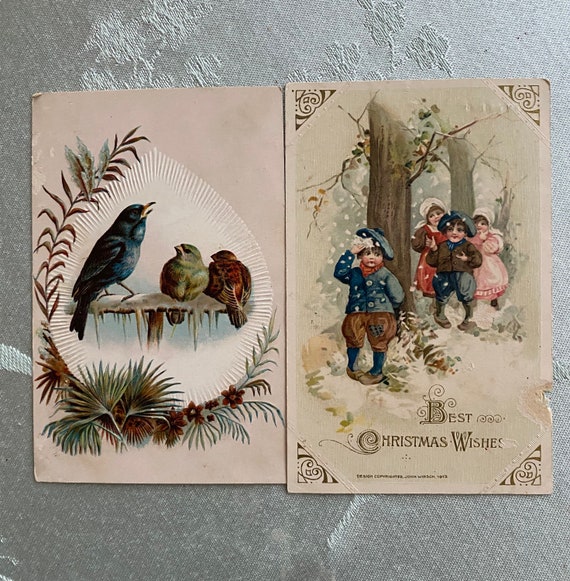The photograph showcases two vintage greeting cards set against an elegantly embroidered white tablecloth. Both cards have a vellum tone, subtly yellowed with age, and exhibit a realistic watercolor painting style. The card on the left features a delicate teardrop-shaped embossed frame displaying a starling and two sparrows, one sparrow facing the starling while the other turns its back to the viewer. This scene is encircled by an intricate garland of leaf fronds, grasses, and nuts. The card on the right offers a festive scene with "Best Christmas Wishes" inscribed at the bottom in an ornate font, with each initial letter lavishly adorned with gold curlicue designs at the corners. The heartwarming image captures a group of cherubic-faced children strolling in the snow under wintry trees—girls in poofy dresses and kerchiefs, boys in knickers and floppy hats—emphasizing the nostalgic charm of the setting.